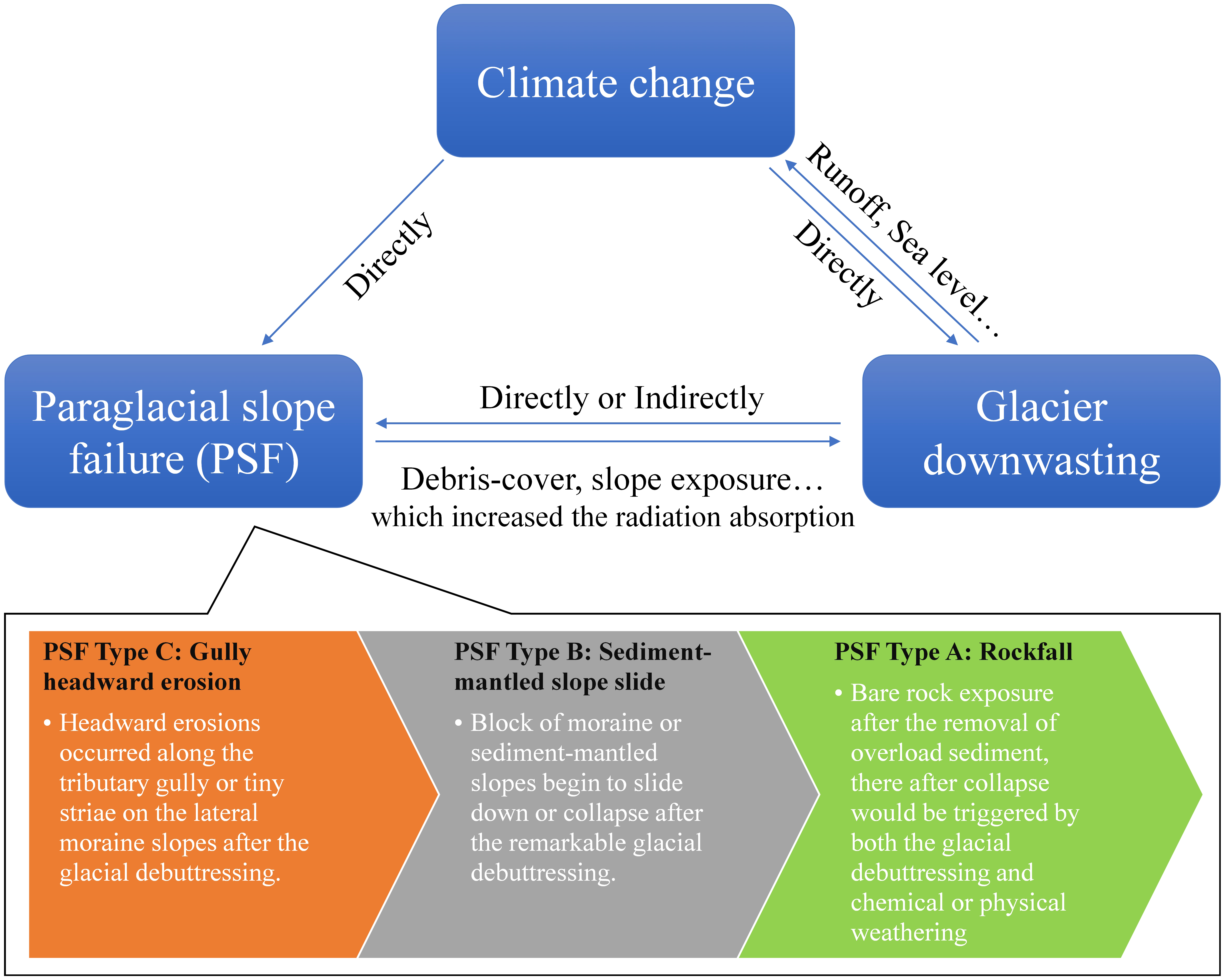The diagram illustrates the interplay between climate change, paraglacial slope failure (PSF), and glacier downwasting on a white background. The rectangular shapes, which are blue with white text, are labeled "Climate Change," "Paraglacial Slope Failure (PSF)," and "Glacier Downwasting." Arrows indicate the direct and indirect relationships among these elements: climate change directly impacts both PSF and glacier downwasting, while PSF and glacier downwasting influence each other reciprocally. Additionally, glacier downwasting contributes to climate change through runoff and sea level changes.

A detailed speech bubble with color-coded sections (orange for PSF Type C, gray for PSF Type B, and green for PSF Type A) elaborates on the different forms of PSF:
- **PSF Type C: Gully Headward Erosion** - Erosions occur along tributary gullies or tiny striae on the lateral moraine slopes after glacial deep attressing.
- **PSF Type B: Sediment Mantle Slope Slide** - Blocks of moraine or sediment mantle slopes begin to slide or collapse post significant glacial deep attressing.
- **PSF Type A: Rockfall** - Exposed bare rock, resulting from the removal of overlying sediment, collapses triggered by glacial deep attressing and subsequent chemical or physical weathering.

This diagram effectively visualizes the complex connections and processes influenced by climate change within glacial and paraglacial environments.